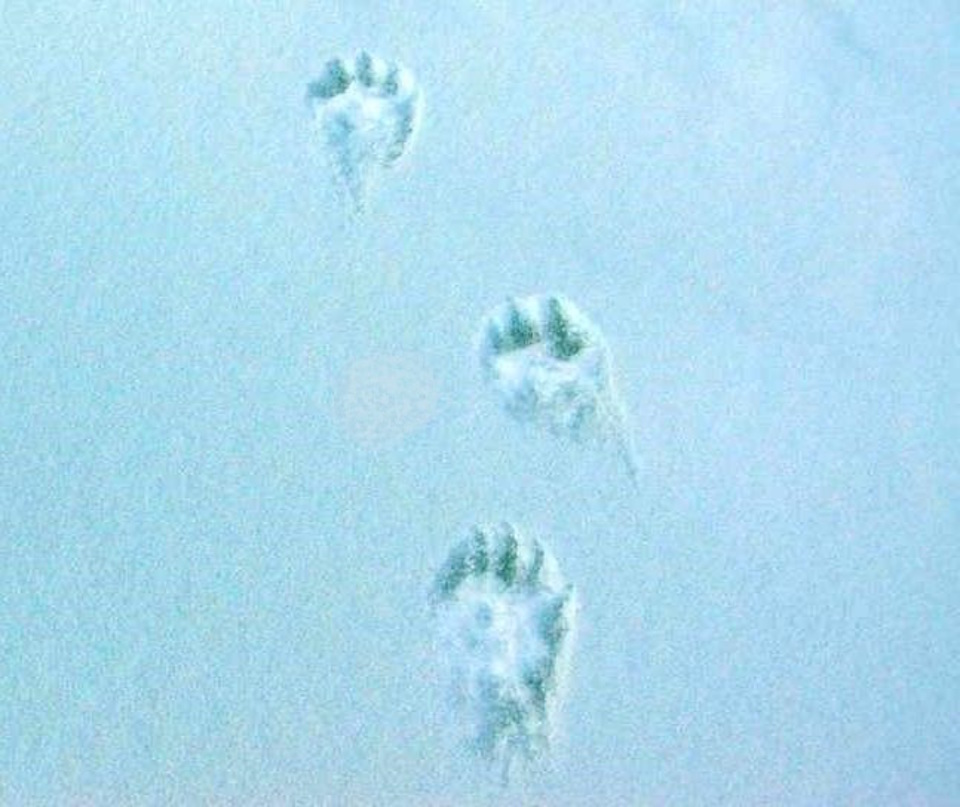This photograph features a close-up of three paw prints embedded in snow, characterized by a grainy texture reminiscent of an old camera. The snow appears bluish-white with a slight yellow tint. The paw prints are spread out, with one at the center bottom, another angled to the left just above it, and a third further up on the left, heading straight up. Each paw print shows distinct triangular claw imprints and rounded toe pads, with roughly three to five claws visible. The largest paw print, closest to the viewer, suggests it was left by a large cat or wolf-like creature. The uniform and pristine snow is interrupted solely by these detailed animal tracks.